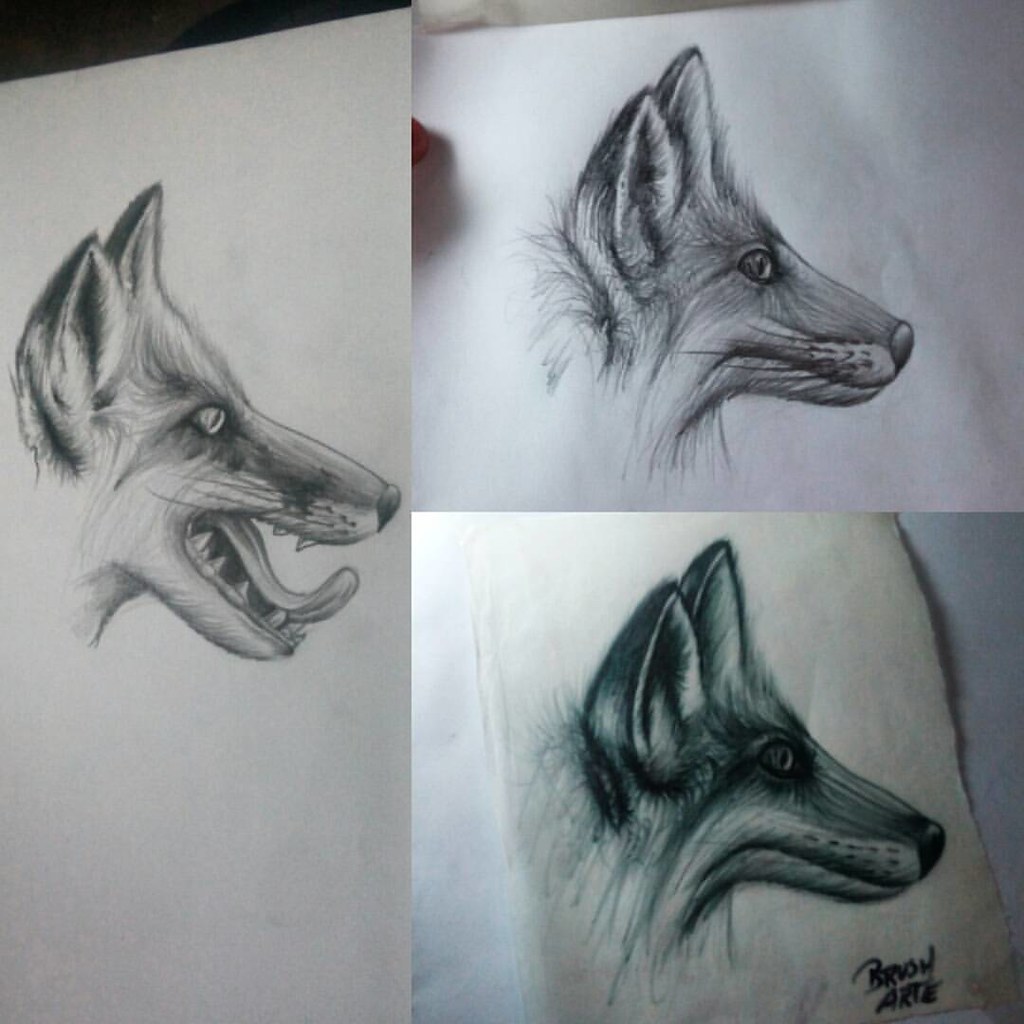This photograph showcases three detailed pencil sketches of a dog's head. The largest sketch spans the entire width of the image, capturing the dog's expressive face with its mouth open, revealing teeth and a curling tongue. The other two sketches are stacked vertically, equally sharing the height space and both depicting the dog with its mouth closed. One of these sketches is signed by the artist, Brian Arte, and in one corner of the image, a finger is subtly visible, holding up the sketch paper.